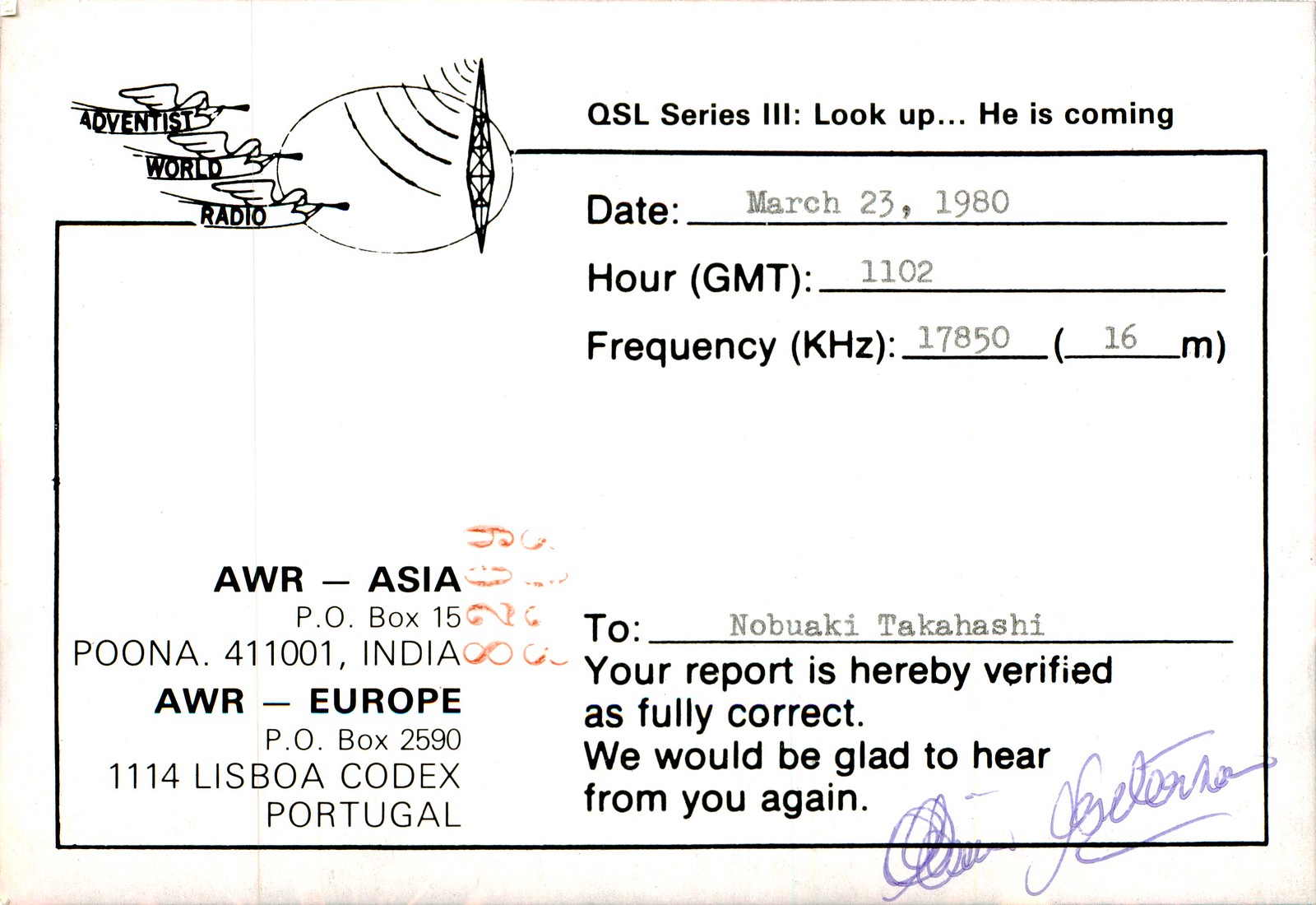The image displays a confirmation receipt from Adventist World Radio, designated as part of the QSL Series 3 with the slogan "Look up, He is coming." Dated March 23, 1980, at 1102 GMT, it verifies a report received on the radio frequency 17850 kHz (or 16 meters). The top features a logo of angels with trumpets flying towards a radio tower. On the left, two addresses are listed: "AWR-Asia, P.O. Box 15, Pune 411001, India" and "AWR-Europe, P.O. Box 2590, 1114 Lisboa Codex, Portugal." The bottom right contains a personalized message to Nobuaki Takahashi, confirming the correctness of the report and inviting future correspondence, followed by a handwritten signature in blue ink.